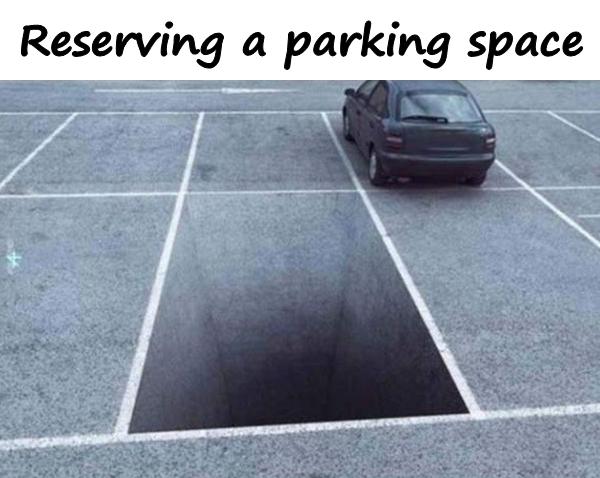A photograph depicts a gray parking lot divided by white lines into numerous parking spaces. Only one dark-colored car is parked in the upper right corner of the lot, its rear facing the viewer with tires visible but no license plate. Above the image, a heading in a dark bluish-purple color reads "Reserving a Parking Space." The largest parking space, situated in the middle bottom area, features a striking optical illusion: it appears to be a deep, dark pit or black hole with side walls, creating the impression that any car attempting to park there would fall through. This cleverly painted illusion ensures that the space visually deters anyone from parking in it.